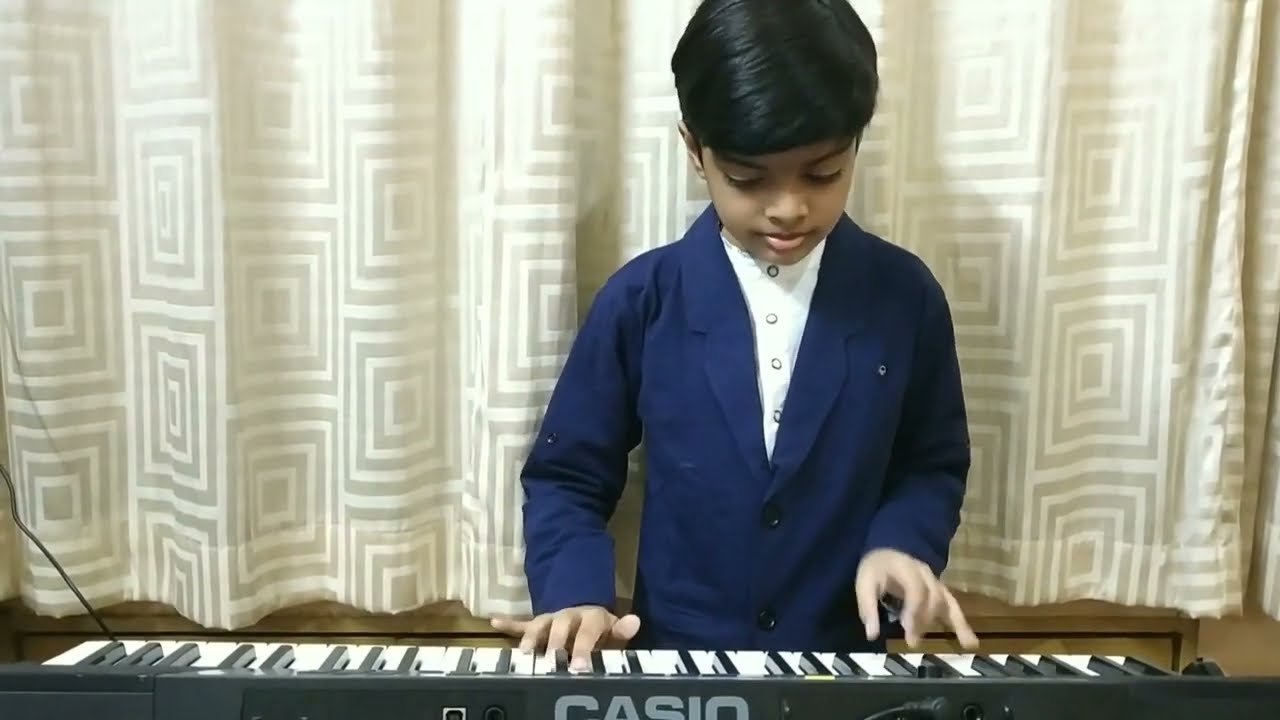The image features a young boy, approximately 7-10 years old, of Indian subcontinent descent, deeply engrossed in playing a Casio keyboard. He is dressed in a white button-up shirt under a smart blue blazer, with his medium-length black hair neatly combed to the side. One hand is pressing the keys, while the other is poised above them, suggesting concentration and engagement. The keyboard, prominent at the bottom of the image, with the Casio brand name visible, contrasts with the boy's small stature, emphasizing the scale of the instrument. The backdrop consists of a curtain adorned with concentric square patterns, rendered in shades of gray over a beige or cream base, adding depth and texture to the high-definition, captivating photograph.